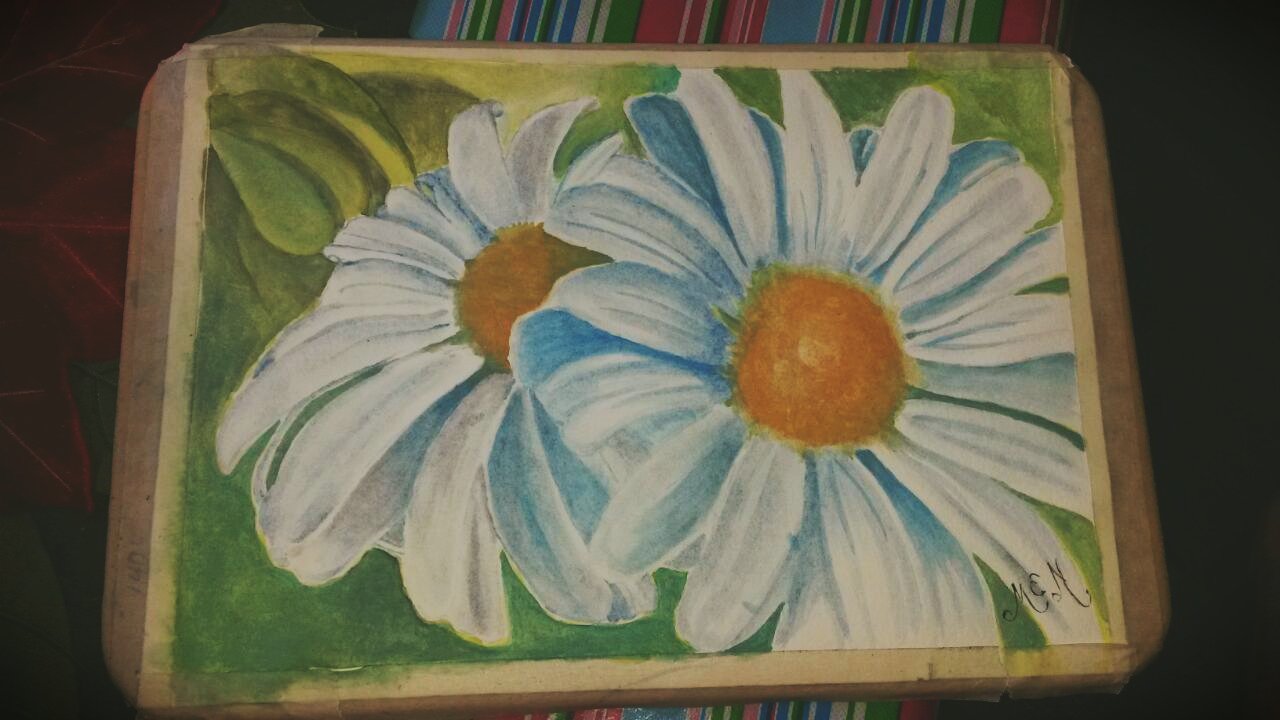This is a highly detailed painting of two large daisies that dominate the scene, both featuring yellow or orange centers and surrounded by about a dozen slightly curved white petals with intricate grooves. The daisy on the right slightly overlaps the one on the left. The painting appears to be done in pastels on a wooden-like surface and is accompanied by a green background with some blue shading. An array of various colors such as blue, pink, green, and white can be found in the background, adding depth and complexity. Additionally, there is a reddish object in the top left corner of the image. The artwork has been signed at the bottom, possibly with the initials "M-E-M" or "M-E-N." The entire painting appears to be placed on a dark surface, enhancing its vivid colors and intricate details.